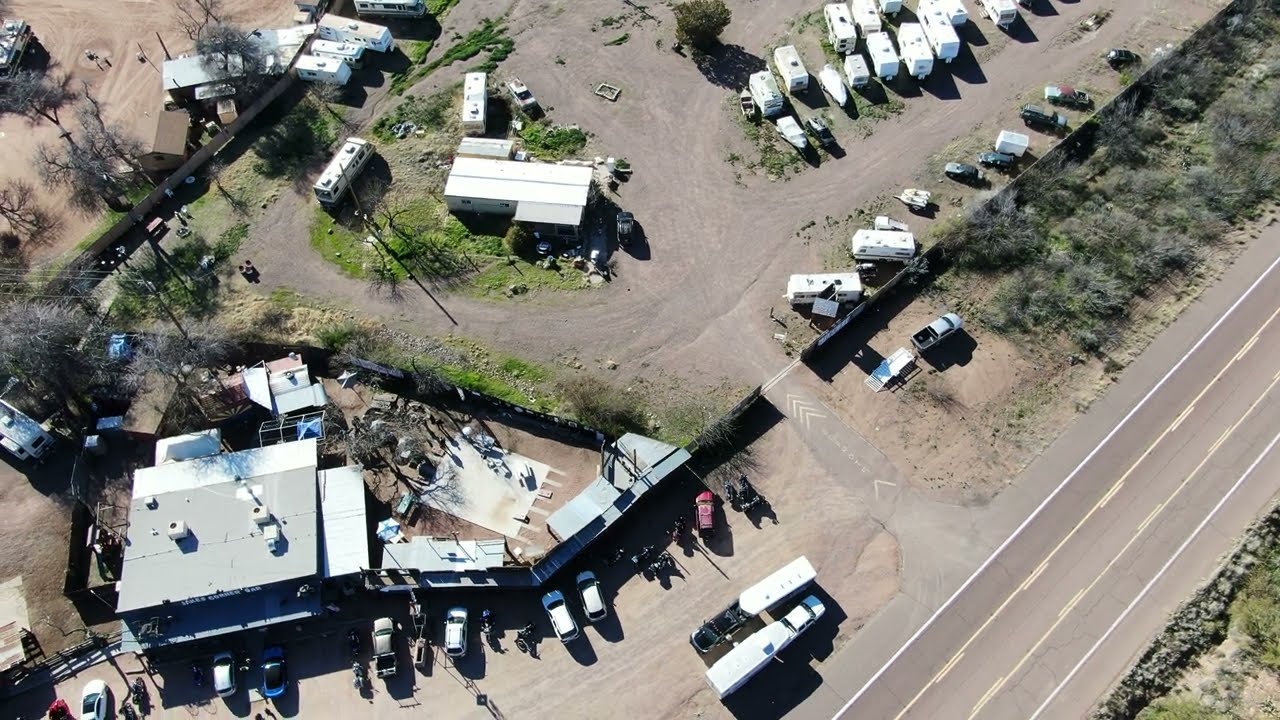The image is an aerial view, likely captured by a drone, showcasing a dusty, expansive area that appears to function as an RV or trailer park. To the top of the image, a large dirt lot is populated with numerous RVs and trailers. The ground is primarily dirt with occasional patches of grass, under a clear, bright daytime sky, suggesting a sunny setting. A two-lane diagonal road intersects the bottom right corner of the image, featuring both solid white and yellow lines, and possibly a bike lane on the right side. Adjacently, there are areas of grass along the road edges. In the lower left corner, there's a business establishment, possibly a bar or restaurant named "James Corner Bar," with several cars parked in front. Additionally, the left side of the image has sandy or dirt patches, and there's a series of black cars that could indicate a passing train. The image distinctly lacks any written words or numbers, emphasizing the outdoor and expansive view of this trailer park area.